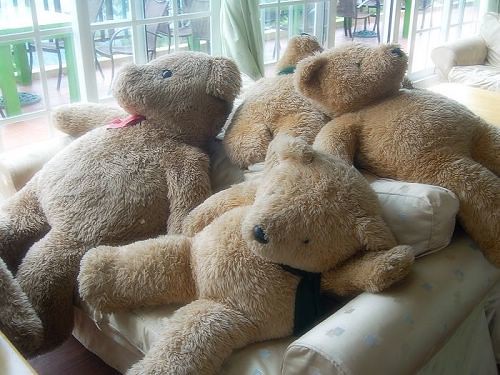In a well-lit indoor setting, this color photograph captures a cozy scene featuring a light-colored fabric couch adorned with four large, coffee-colored teddy bears. The bears, each with black button eyes and noses, are arranged in a relaxed, haphazard pile, mostly looking outward. The couch, either pale green or white with a subtle pattern, anchors the image while a wall of large windows in the background floods the room with natural light. Visible through the windows are buildings, vegetation, and hints of outdoor furniture made of black wrought iron. Adding a splash of color to the neutral-toned bears, one sports a blue neckerchief, and another a red one. The light wood flooring adds to the airy ambiance of the room.